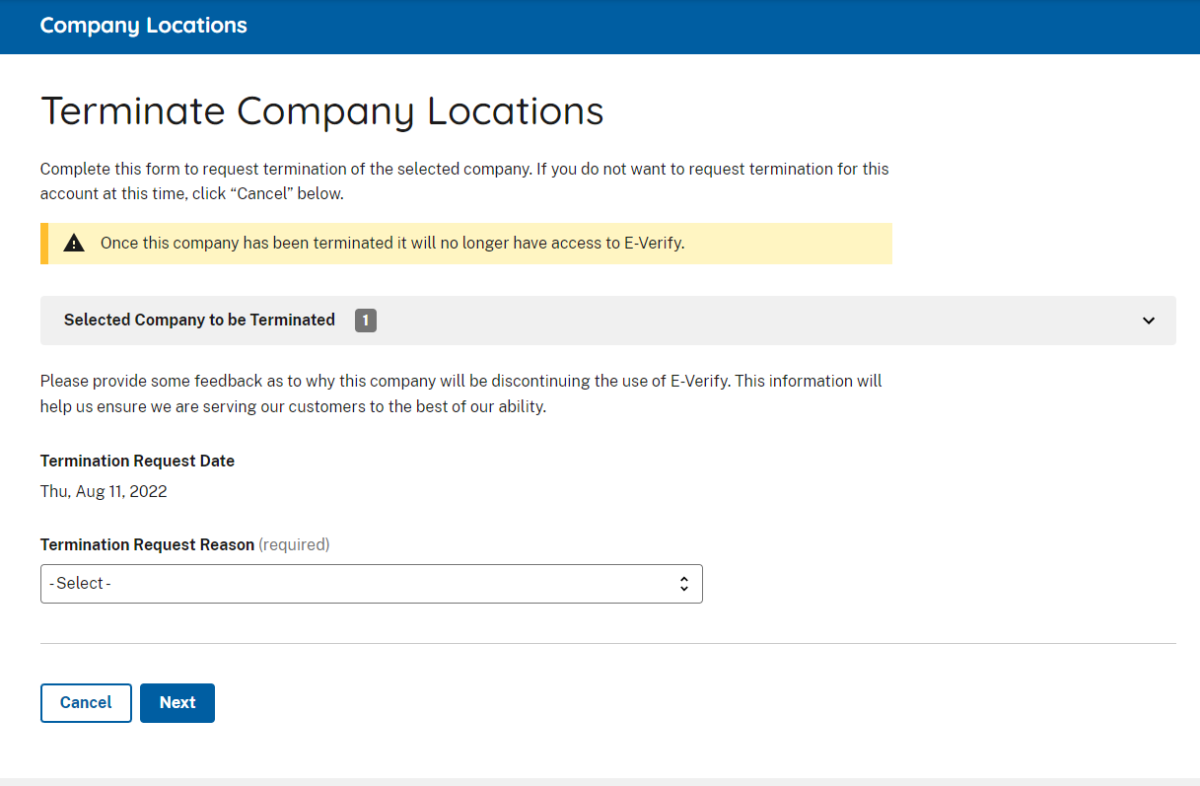This is a detailed screenshot of a company website's 'Location Termination' page. At the top left corner, a blue horizontal bar spans the full width of the page, featuring the text 'Company Locations' in white, with both 'C' and 'L' capitalized. Directly below this, the phrase 'Terminate Company Locations' appears in black font against a white background. Beneath these headers, the instructions 'Complete this form to request termination of the selected company. If you do not want to request termination for this account at this time, click Cancel below,' are displayed in clear black text. A yellow notification bar below the instructions reads, 'Once the company has been terminated, it will no longer have access to eVerify.' Under this, there is a section titled 'Selected Company to be Terminated.' This section includes a gray box with the number '1' inside it. Finally, at the bottom, the termination request date is specified as Thursday, August 11, 2022.